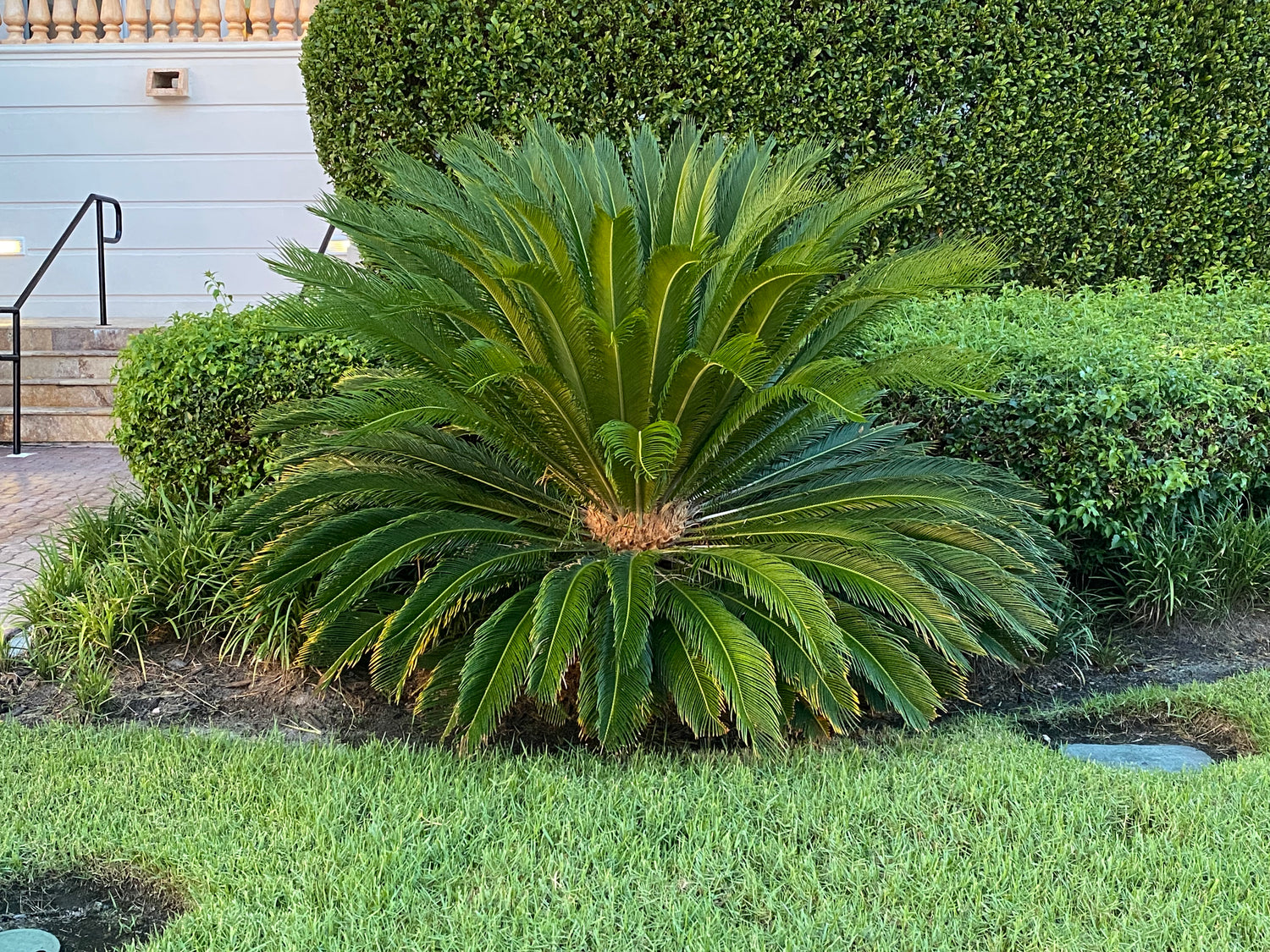This outdoor image showcases a landscaped area dominated by a unique short palm tree. The tree features a shaggy, light brown trunk visible between two distinctive bunches of long, skinny fronds. The first bunch fans out horizontally around the base, while the second cluster arches upward in various directions, culminating in orange-pinkish hues at its center. Surrounding this central palm are several well-manicured bushes and hedges, including a large bush in the background, all situated within a mulched area. The foreground is occupied by a lush, green lawn, though there are a few bare patches, one revealing a flat stone and another possibly exposing a sprinkler mechanism. On the top left of the image, a tan-colored staircase with four steps and black railings leads up to a paver driveway and the wall of a building, creating a structured backdrop to this serene outdoor scene.